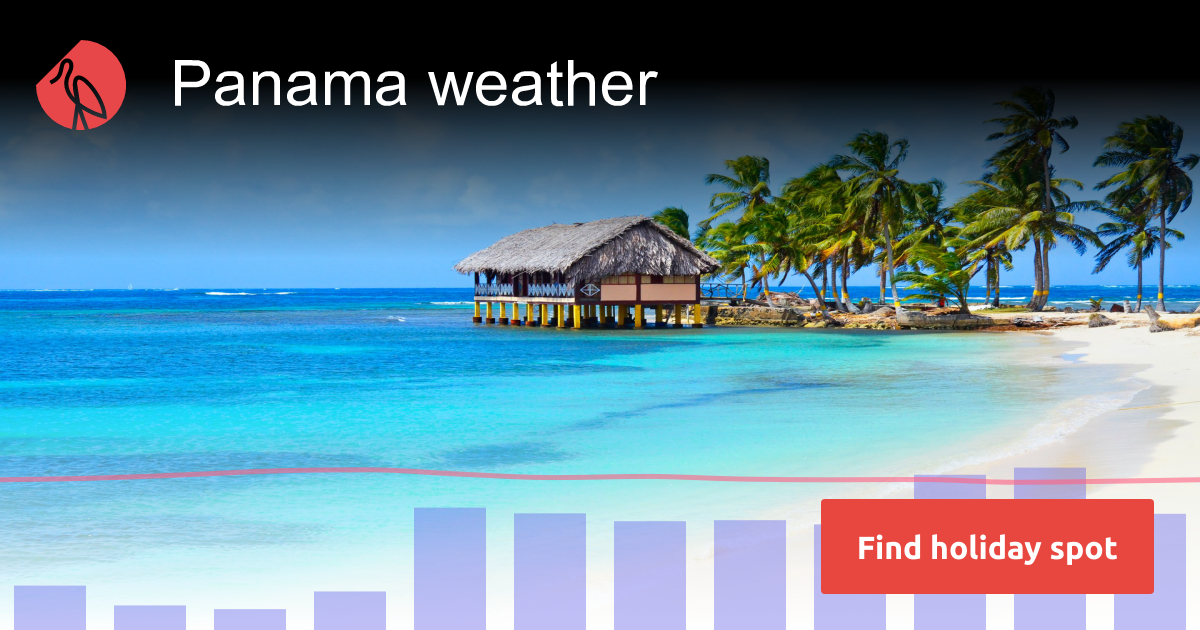This is a screenshot of a website named "Panama Weather". At the top, the title "Panama Weather" is prominently displayed in large white letters. To the right of the title, there is a logo featuring a red circle with a black line drawing of a flamingo inside. The title "Panama Weather" is positioned within a black banner that gradually fades into a static background image covering the entire page.

Beneath the banner, there is a bar graph superimposed onto the background image. The bars extend from the left side to the right side of the screen, starting small, gradually increasing in size, and culminating in very large bars towards the end. A red line runs across the top of the graph, and the two bars on the far right reach up to touch this red line.

In the bottom left corner of the screen, there is a prominent red box with the text "Find Holiday Spot" written in white.